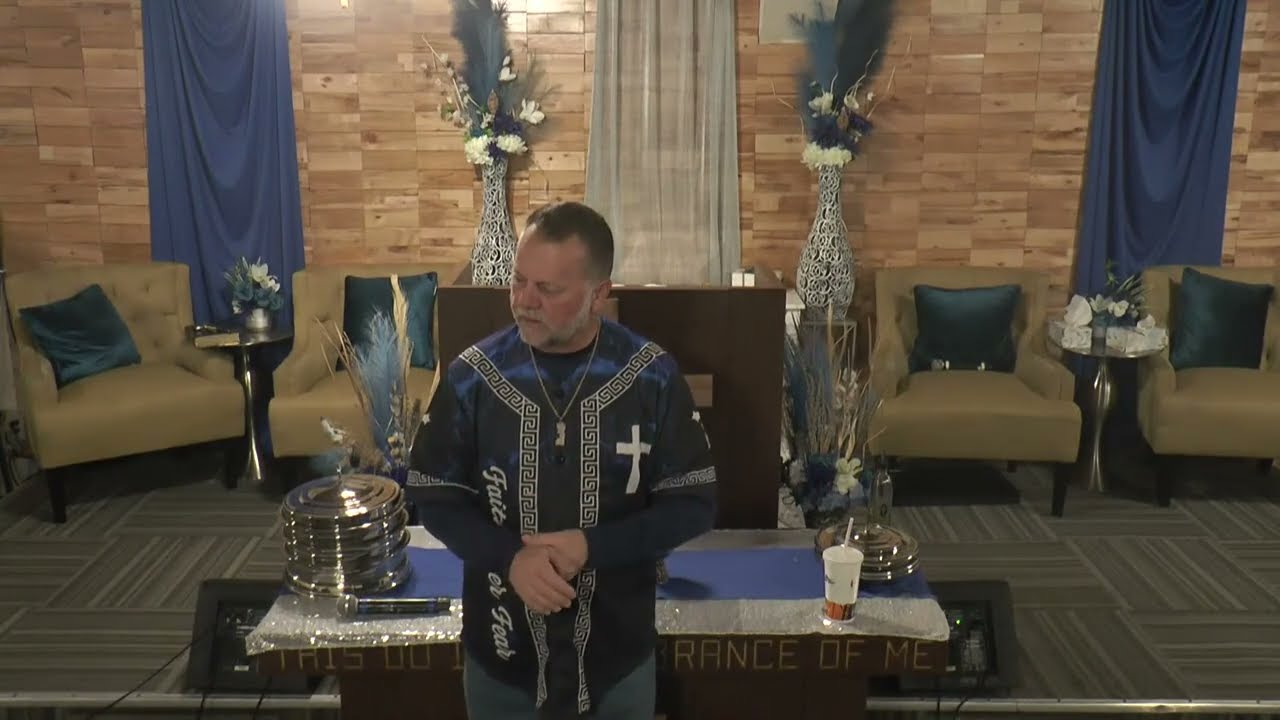The image depicts a religious setting, possibly within a church or mosque, featuring a person clad in a distinctive blue robe-like shirt. The shirt is medium to dark blue with a tie-dye pattern and features white and black or blue borders running down from the shoulders to the waist, where a white cross is prominently displayed. The long-sleeved garment has text in white that reads "faith something" and repeats the word "faith." The person, who may be a religious leader like a pastor or preacher, stands with arms clasped in front of a brown altar adorned with a blue table runner.

On the altar, a variety of items are present: communion plates, a microphone, and incongruously, a McDonald's drink cup, which disrupts the otherwise sacred atmosphere. The altar is set against a background of a brick or wooden-paneled wall with blue and possibly clear or white drapes. Beige chairs line the area, and decorative blue and white vases filled with white flowers are placed nearby. This setting exudes a casual yet devout ambiance typical of some religious venues.